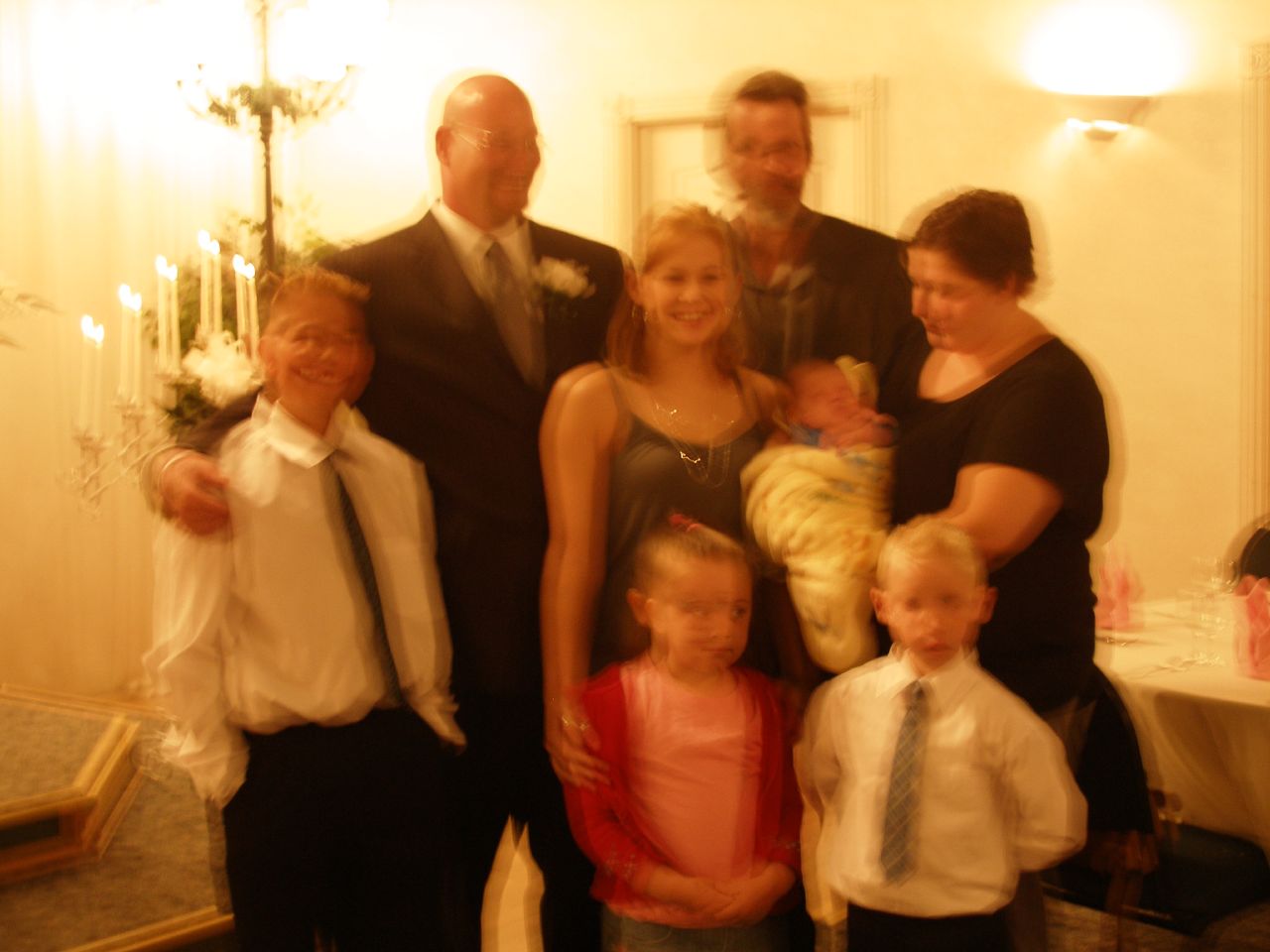This color photograph is incredibly blurry but appears to depict a family gathering, possibly in a church, dining hall, or at a wedding. The image shows eight individuals dressed formally. The central figure in the back is a bald, larger man with round metal-rimmed glasses and a short beard and mustache. He is wearing a black tuxedo with a white undershirt, a gray tie, and a white corsage pinned to his right pocket. He has his arm around a man in the front row who is dressed in a white dress shirt, black tie, and black pants. This man has dirty blonde hair.

To the right of the bald man is a woman in a gray strapped dress, wearing silver necklaces, and smiling for the camera. She has long blonde hair and is holding an infant wrapped in a white blanket with blue accents in her right arm. The infant has a blue shirt and a small amount of brown hair. In front of the woman, there are two children: a girl with a red bow in her dirty blonde hair, wearing a red jacket over a pink shirt and blue pants, and a boy with blonde hair, wearing a white dress shirt with a blue-and-white striped tie and black pants.

Another woman, helping with the infant, stands next to the woman in the gray dress. She has short brown hair, a short-sleeved black shirt, and is looking at the baby. The last individual, on the far right, has short brown hair, a salt-and-pepper beard, and is wearing glasses and a dark gray shirt.

Behind the group, there are lit white candles that might be part of a menorah, suggesting a religious or festive setting. The candles have a white flame, and additional light fixtures can be seen in the background. The lower-left corner of the image reveals what seems to be carpeted stairs or a platform. The scene is adorned with white or cream-colored walls and a white table with pink napkins on plates. Despite the extensive blurriness, the family appears to be celebrating and dressed in their finest attire.